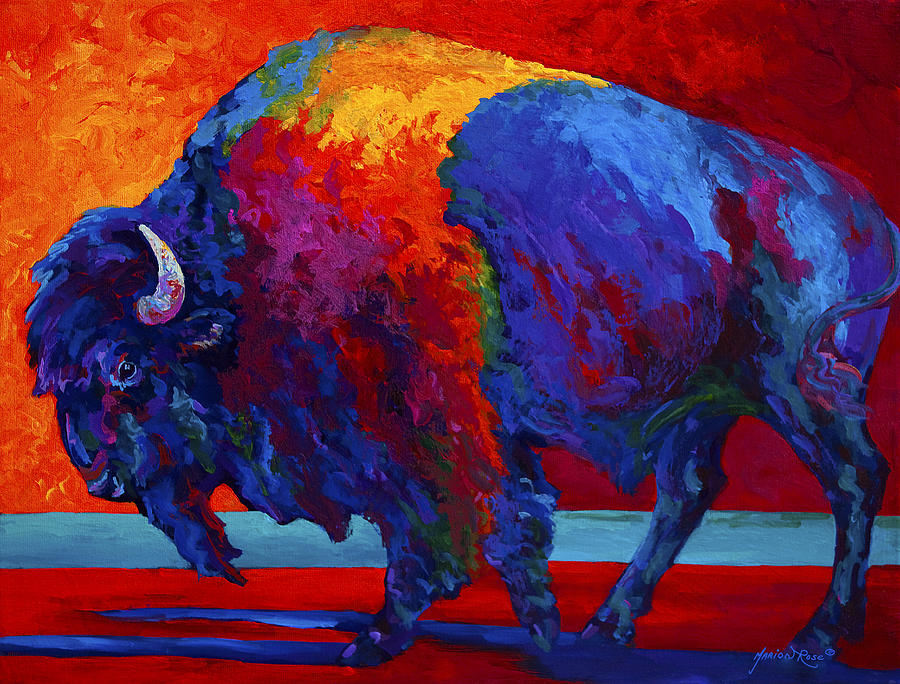This artwork is a striking, technicolor painting of an American bison, or buffalo, predominantly using shades of blue with splashes of red, orange, yellow, and hints of green. The head of the bison is on the left side of the painting, with its back extending to the right. The creature's head, distinctly downturned as if gazing at the ground, showcases a white horn adorned with streaks of red and a black eye and nostril. A small blue beard adds detail beneath the bison's muzzle. The bison's broad shoulders and distinctive hump transition into its back, which is a mix of blue with interspersed red streaks.

The background is a vivid gradient, with the left side awash in orange and transitioning to a deeper red on the right. Below the bison, a surface of red ground is shadowed in blue, suggesting depth and dimension. The lower part of the image includes a blue area, possibly indicating water, creating a contrasting coolness against the warm hues above. The bison is standing tall, its tail swishing to the left, caught mid-air. The composition is further detailed by the artist's distinctive signature in the bottom right corner, affirming the piece’s authenticity. Overall, the vibrant, non-traditional colors and dynamic composition make this painting an eye-catching, abstract representation of the majestic American bison.